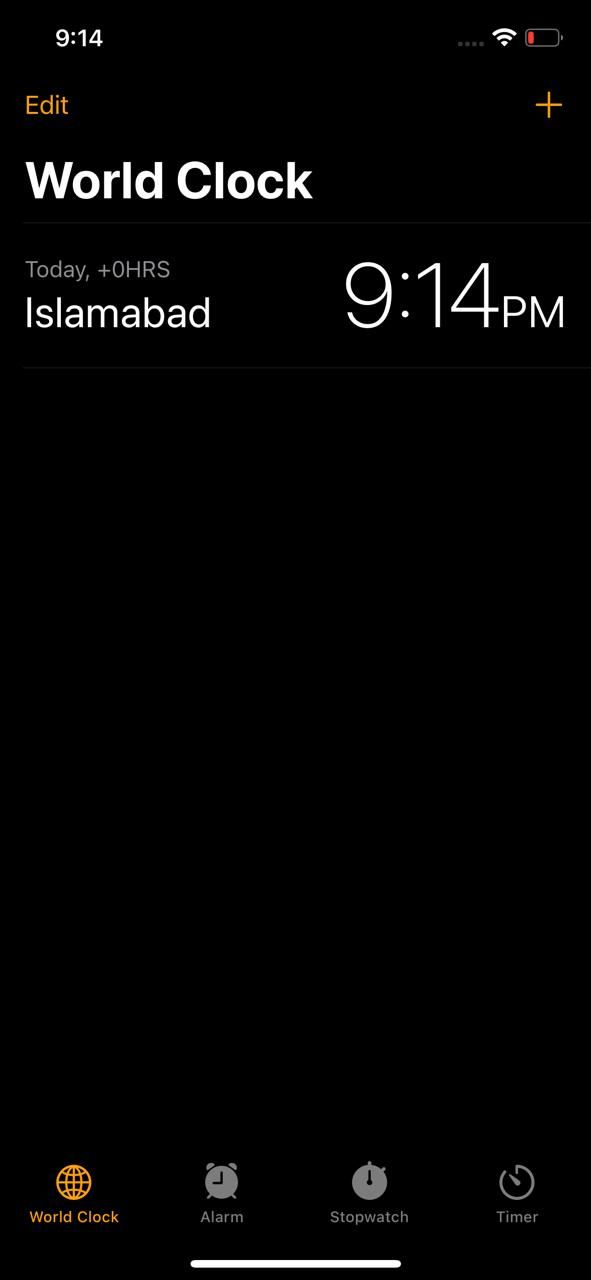This detailed caption could be used to describe the image accurately:

---

"A screenshot from an Apple iPhone's World Clock page, captured at exactly 9:14 PM. The screenshot showcases the time in Islamabad, indicating that it is also 9:14 PM there, suggesting that the user is currently located in Islamabad. No additional world clocks have been set up, focusing solely on Islamabad's time zone. The phone is connected to WiFi but is running critically low on battery. At the bottom of the screen, various icons for alarm, stopwatch, timer, and World Clock are visible. The World Clock icon is highlighted in gold, while the remaining icons are displayed in a muted grey, blending into the background. In the top right corner, a '+' sign is present for adding more time zones, and an 'edit' symbol is located in the top left corner for customization."

---